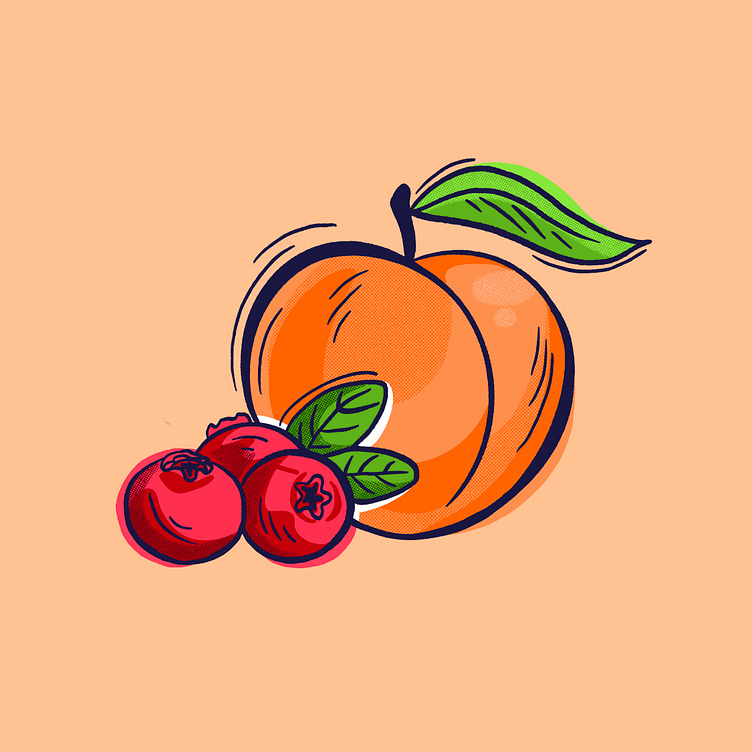This vibrant illustration depicts a ripe, plump peach with a distinctive heart shape and a prominent crease in the middle, accentuated by dynamic lines that suggest movement. The peach is a rich peachy orange color, with a single green leaf sprouting from its stem. Beside the peach are three deep red fruits, possibly raspberries, cherries, or blueberries, each bearing two green leaves. These fruits are round with frilly star-shaped ends, contributing to their unique appearance. The entire scene is set against a light orange, peach-colored background, with a digital painting style that lends an oil painting-like texture and depth to the fruits and their vivid colors.